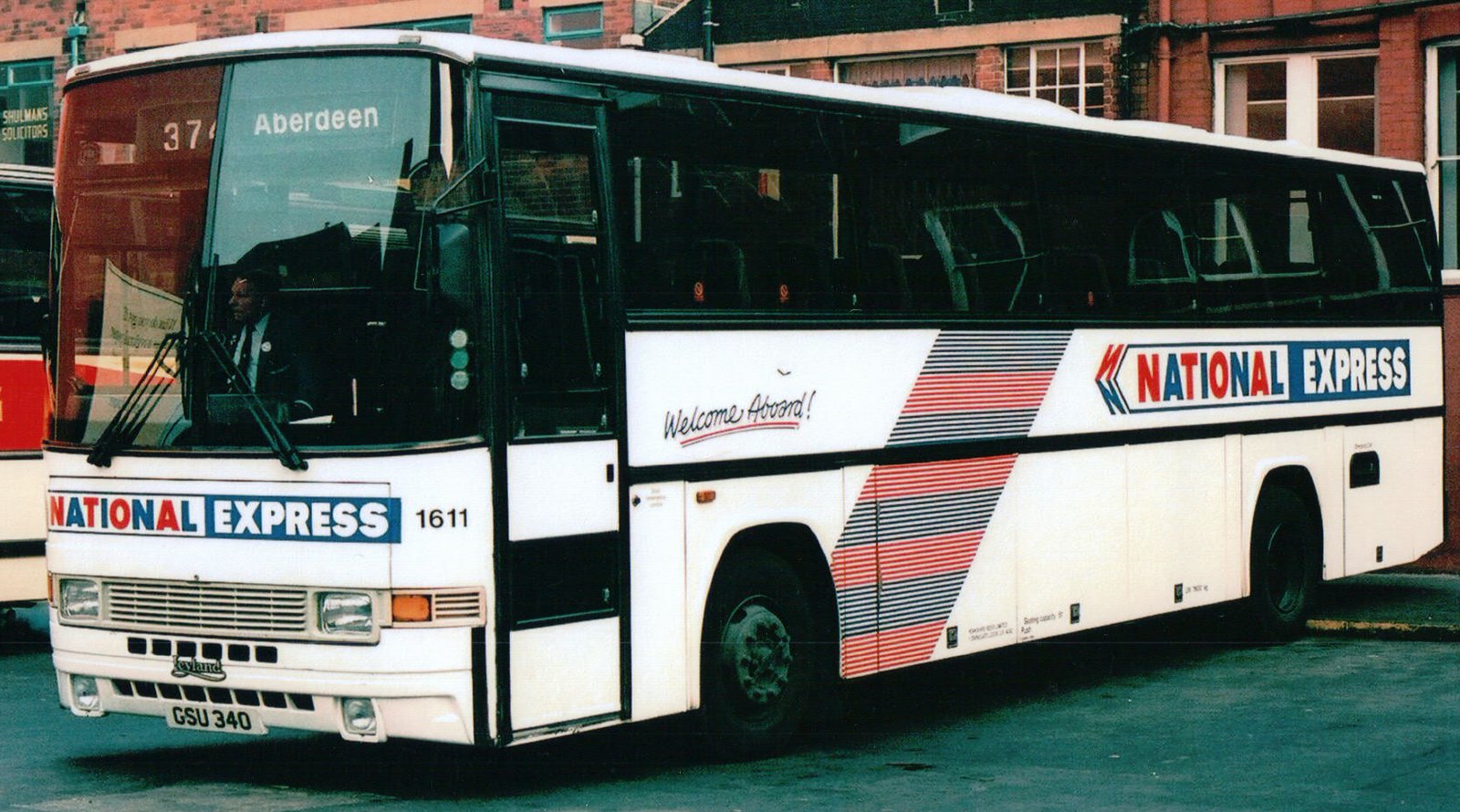A large, predominantly white National Express bus is parked on the pavement in front of multi-story brick buildings that are split into sections. The bus features a mix of blue, red, and black colors and has a flat front design. In multi-colored letters, "National Express" is displayed on both the front and the side of the bus. The sign inside the front windshield reads "37 Aberdeen." Below the windshield, on the bumper, the text "Leyland GSU 340" can be seen. The bus is fairly long and has a passenger door on the side beside the text "Welcome Aboard." Notably, there are large stripes made up of smaller stripes in red and blue adorning the sides. Through the front windshield, the driver is visible, seated in the driver's seat. The brick buildings serve as the backdrop, creating a contrast with the vibrant bus colors.